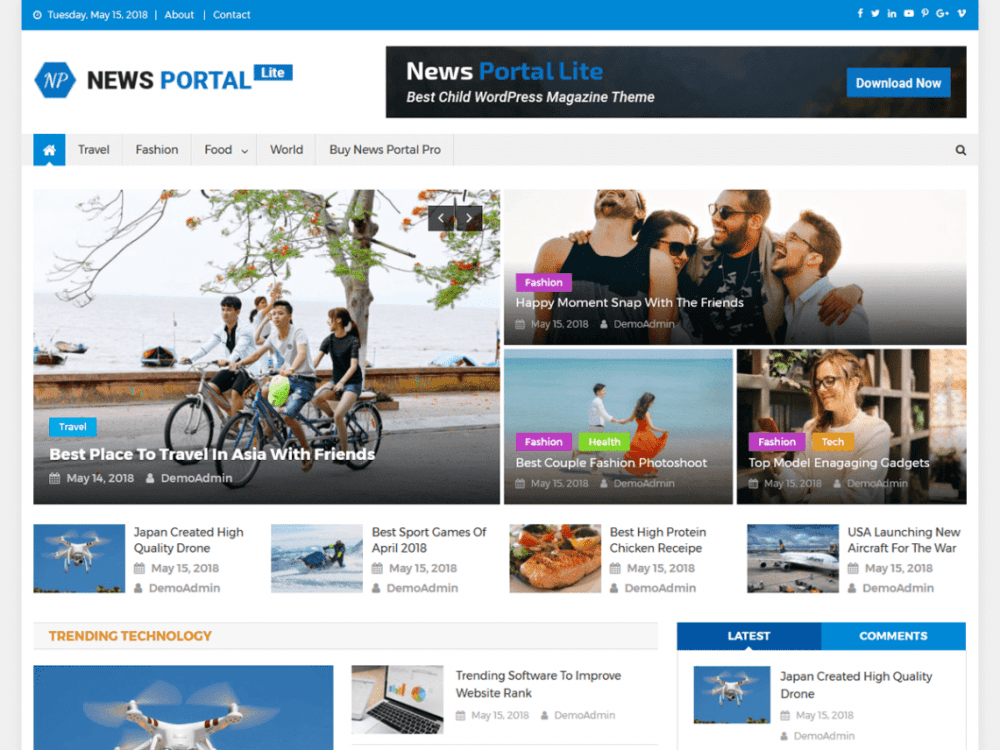The webpage header displays a blue banner with the date "Tuesday, May 15, 2018" prominently featured. On the right side of the banner, there are links labeled "About" and "Contacts," along with icons for various social media platforms such as Facebook, Twitter (now X), LinkedIn, and others that are not clearly identifiable.

The webpage is titled "News Portal Lite" and features a logo consisting of the initials "NP" on a blue background. Adjacent to this is a black banner with white text stating "News Portal Lite," where "News" is in white and "Portal Lite" is in blue. Below this, in white text, it reads "Best Child WordPress Magazine Theme," and there is a prominent "Download Now" button to the right.

Underneath this banner, there are menu options for different categories including Travel, Fashion, Food, World, and a promotional link for "Buy News Portal Pro." Each category is accompanied by an image. 

The "Travel" section displays an image of three people riding bicycles on a street next to a body of water with boats in the background and a tree off to the side. Adjacent to the Travel section, there is an image depicting four people in a close group. One man has his arm around two others, and there appears to be a woman nestled between one of the men and another woman. All four individuals are laughing and wearing some form of eyewear, giving off a sense of joy and camaraderie.